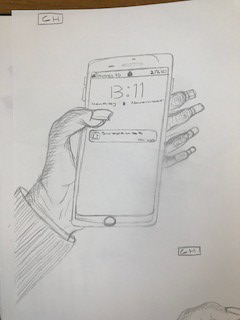This artwork is a detailed drawing of a person's left hand grasping a large cell phone. The phone screen displays the time "13:11," and there appears to be a notification icon near the top, though the exact details are unreadable. The hand is depicted with a thumb resting on top of the phone, sporting a long nail, while the other nails on the hand appear long and somewhat scraggly. In the upper left-hand corner of the image, the initials "GH" are prominently displayed, possibly indicating the artist's signature. The drawing is meticulously crafted, capturing the textures and nuances of both the hand and the phone.